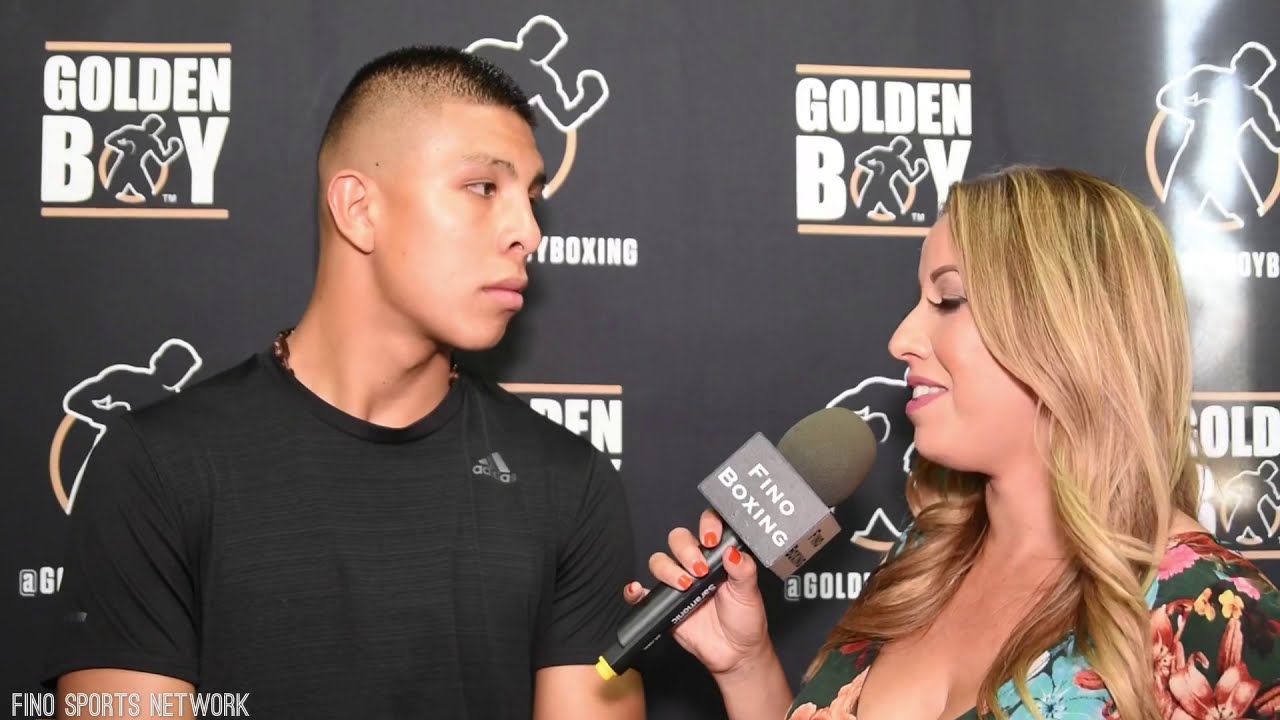The image is a screen grab from an interview at a press conference for Golden Boy Boxing. In the background, there's a repeating press banner with "Golden Boy" and "Golden Boy Boxing" logos, featuring a gold 'O' with a silhouette of a boxer. On the left side stands a young man with light brown skin and very short, almost military-style dark brown hair, shaved on the sides. He is wearing a black short-sleeved Adidas shirt, looking attentively at the interviewer. The interviewer is a woman in her early 30s with long, blonde hair straightened and curled at the ends. She has light brown skin and is wearing a colorful floral blouse. She holds a microphone labeled "Fino Boxing" in her right hand, with orange painted fingernails, and appears to be mid-sentence with her eyes partially closed and mouth open, showing her teeth in a downward-turned smile. In the lower left corner of the image, a watermark reads "FINO Sports Network."